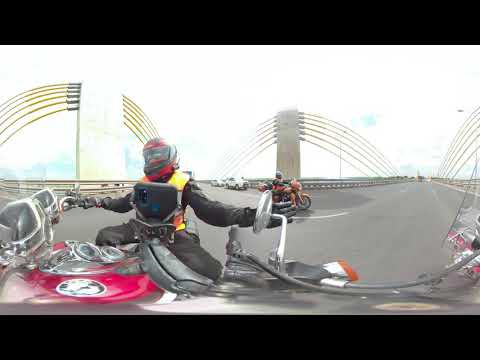In this intriguing photograph, a man standing beside a vividly red motorcycle is prominently featured against a distorted yet captivating backdrop. He is dressed in a black motorcycle jacket and pants with a red helmet featuring a black visor. The motorcycle, primarily red with black accents, appears exaggeratedly stretched due to the image's distortion, giving the impression that his arms are spread wide as he grasps the handlebars. The stretching of the image also affects the surrounding structures, creating an arch-like or semi-circular visual frame, possibly composed of asphalt streets and interstates with white lines or steel rods forming part of an overpass.

To his left, behind his helmet and black-gloved hand, the highway extends into the distance, appearing more natural and undistorted. Here, another motorcyclist can be seen riding away along with several cars in the background. The entire scene is bordered by thick black strips at the top and bottom, adding to the sense of compression and convolution. Framing the man and his bike is a mix of normalcy and visual warp, contrasting sharply with the surreal, almost optical illusion created by the elongated figures and road structures. The sky, tinged with hues of white and blue, softly crowns the complex and detailed landscape of this highway tableau.